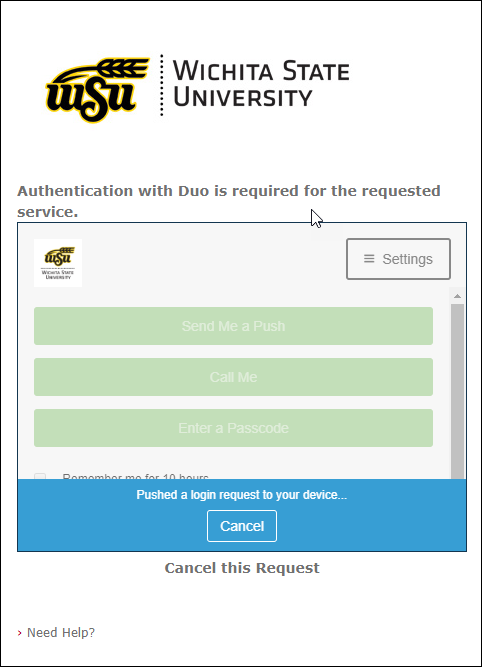This screenshot from Wichita State University's website captures a login page that requires Duo authentication. On the left side, the WSU icon prominently displays "WSU" in black letters outlined in gold. The primary instruction reads: "Authentication with Duo is required for the request to the service," indicating that Duo must be used to proceed.

A darker gray border frames the main content area, which features several options in a light gray background. Three green horizontal buttons present the options: "Send Me a Push," "Call Me," and "Enter a Passcode." Below these options sits a blue bar with instructions: "Push the login request to your device," accompanied by a cancel button labeled "Cancel" in white text.

Lower down on the page, a white section labeled "Need help?" sits on the left, along with a gray question mark in handwriting style. Additionally, there is an option to "Remember me for 10 hours" located beneath the green Duo authentication buttons. Overall, the page is designed to be straightforward and user-friendly.